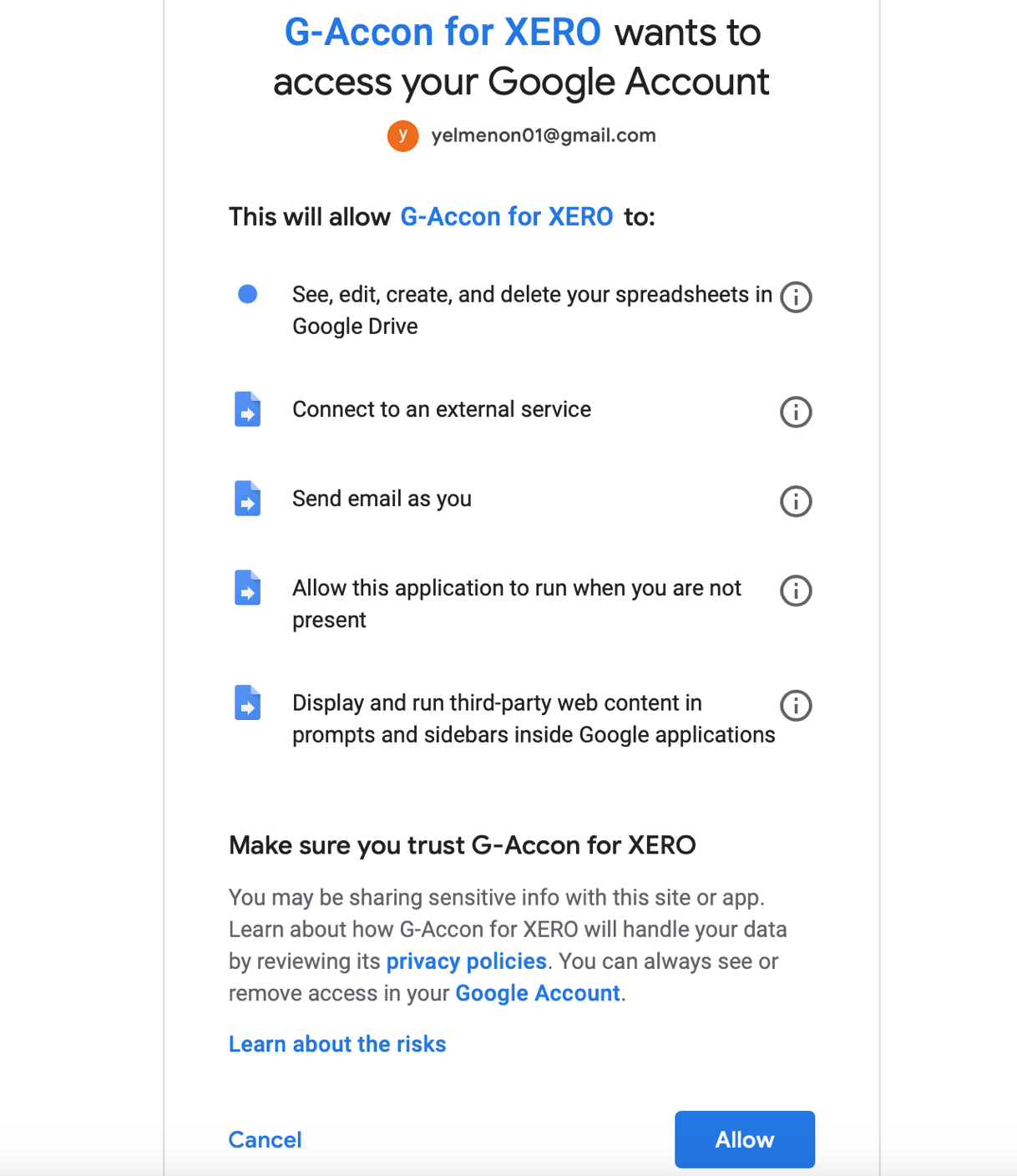The image displays a Google authorization page where an application named "GACCON402" is requesting access to a user's Google account. At the top of the page, in bold black text, a message reads: "GACCON402 wants to access your Google account." Beneath this message, the user's email address is displayed prominently. 

The permissions being requested by "GACCON402" are detailed, including the ability to view, edit, create, and delete Google Spreadsheets in Google Drive, connect to an external device, send emails on behalf of the user, run applications in the user's absence, and display and run third-party web content and scripts in Google applications. 

At the bottom of the page, a cautionary note advises users to only proceed if they trust the application, as they could be sharing sensitive information. There are links providing additional information about data handling and privacy policies, all rendered in blue text. 

The page's layout is clean and minimalistic, featuring predominantly white background with black text, and small blue icons representing documents next to some of the listed permissions.